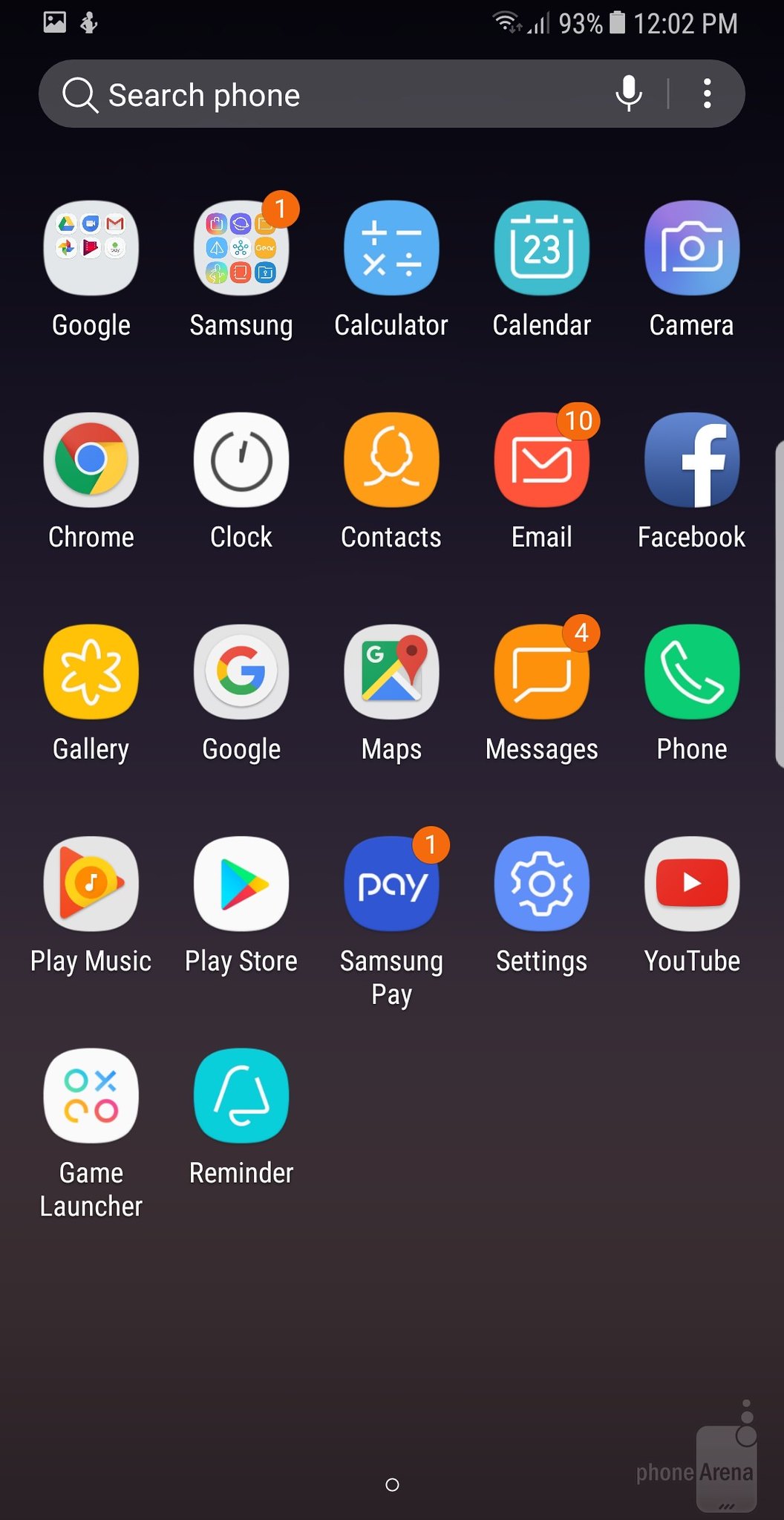This image is a detailed screenshot of a smartphone's home screen, displayed with a black background and pale white text. At the very top of the screen, there is a status bar featuring a landscape photo mode icon, a fitness tracker icon with a woman running, a Wi-Fi indicator, a 93% battery icon, and the current time, which is 12:02 PM. Beneath these elements, there is a search bar labeled "Search phone" accompanied by both a magnifying glass icon and a microphone icon for voice-to-text inputs.

The home screen is divided into five rows of app icons and widgets. The top row includes:
1. A Google cluster with icons for Google Drive, Gmail, Google Play, and several other Google apps.
2. A Samsung cluster housing various Samsung apps.
3. Separate icons for Calculator, Calendar, and Camera.

The second row comprises:
1. Chrome.
2. Clock.
3. Contacts.
4. Email (notably featuring an orange circle with the number 10, indicating unread messages).
5. Facebook.

Following that, the third row includes:
1. Gallery.
2. Google.
3. Maps.
4. Messages (with four new messages indicated).
5. Phone.

The fourth row is made up of:
1. Play Music.
2. Play Store.
3. Samsung Pay.
4. Settings.
5. YouTube.

Finally, the bottom row contains only two icons:
1. Game Launcher.
2. Reminder.

Overall, the screen is well-organized, showcasing a blend of essential apps and frequently used services for quick access.